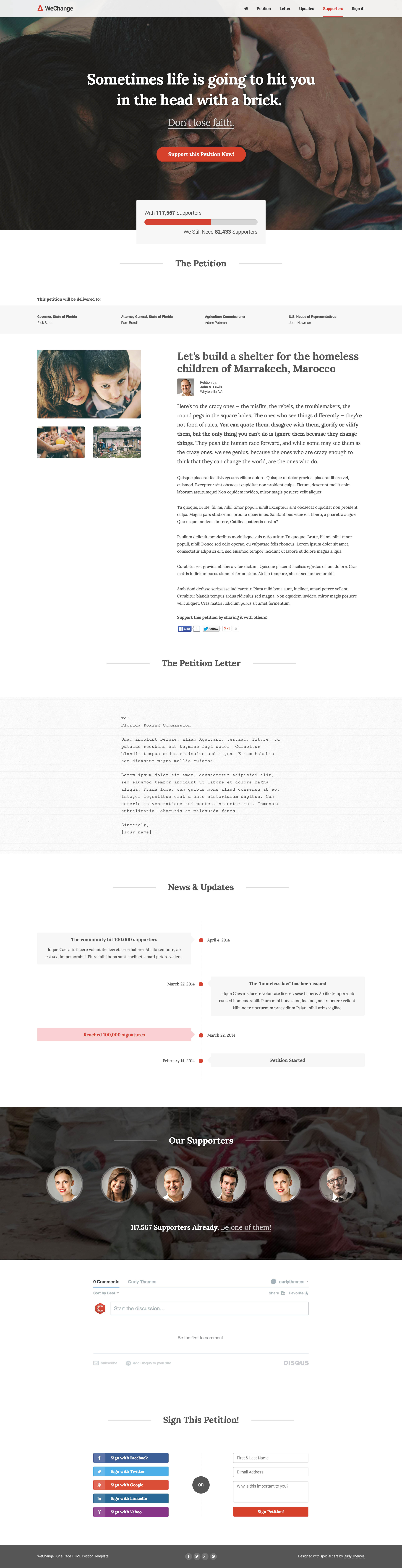In this time of crisis, we unite for change. Join us in supporting this crucial petition by signing and sharing it. Currently, we have 117,567 supporters, but we need an additional 82,433 to reach our goal. This petition, when fully supported, will be delivered to the Governor of Florida, Rick Scott; Attorney General, State of Florida, Pam Bondi; Agricultural Commissioner, Adam Putnam; U.S. House Representative, John Newman; and Petitioner, Rick Scott. Remember, life can hit you hard, but don't lose faith—stand with us and make a difference.